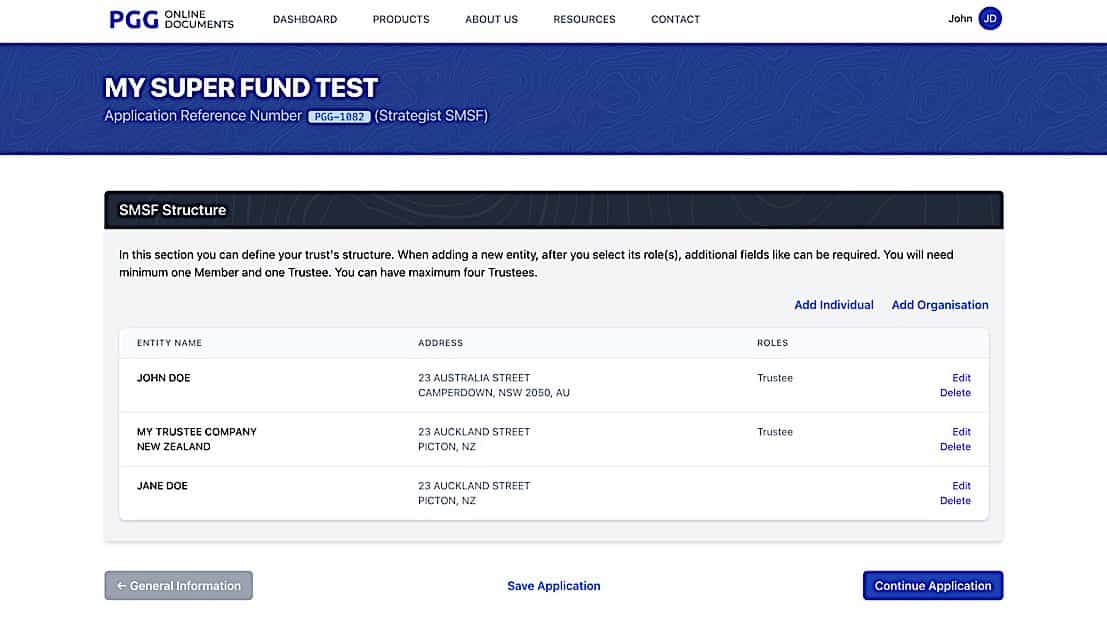The image is a screenshot of a website displaying general information. The top left corner features a title that reads "PGG Online Documents." Below the title is a subheading stating "My Super Fun Test," followed by "Application Reference Number: PGG-1882." The section titled "SMSF Structure" provides guidelines for defining a trust structure when adding a new entity. It explains that after selecting roles, additional fields may be required. A minimum of one member and one trustee is necessary, with a maximum allowance of four trustees. The section also includes various addresses and examples for reference.